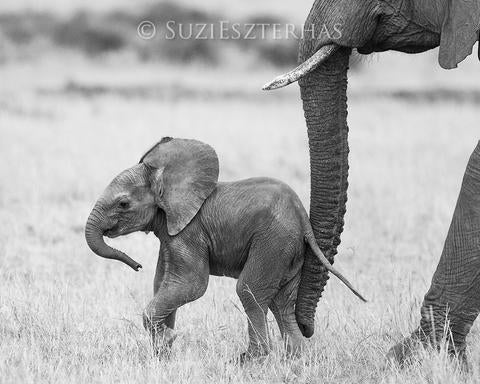This detailed black-and-white photograph, watermarked by Suzie Szterhas, captures the tender moment of a mother and baby elephant journeying across a grassy savanna. The baby elephant, the focal point of the composition, is positioned in the center bottom of the photo, confidently walking with its trunk curved towards its body and its ears back. Notably, the baby elephant does not yet have tusks. Surrounding the youngster, the tall grasses of the prairie add texture to the image, adding a sense of their natural environment.

In the background, gentle hills painted in shades of grey suggest a calm day under open skies. Meanwhile, the mother elephant, partially visible on the right side of the image, offers a protective presence. Only her trunk, guiding the baby’s back leg, along with a single tusk, part of her ear, and one front leg are seen. This image encapsulates the bond between the mother and her young as they traverse their habitat, a serene and timeless moment immortalized in monochrome.